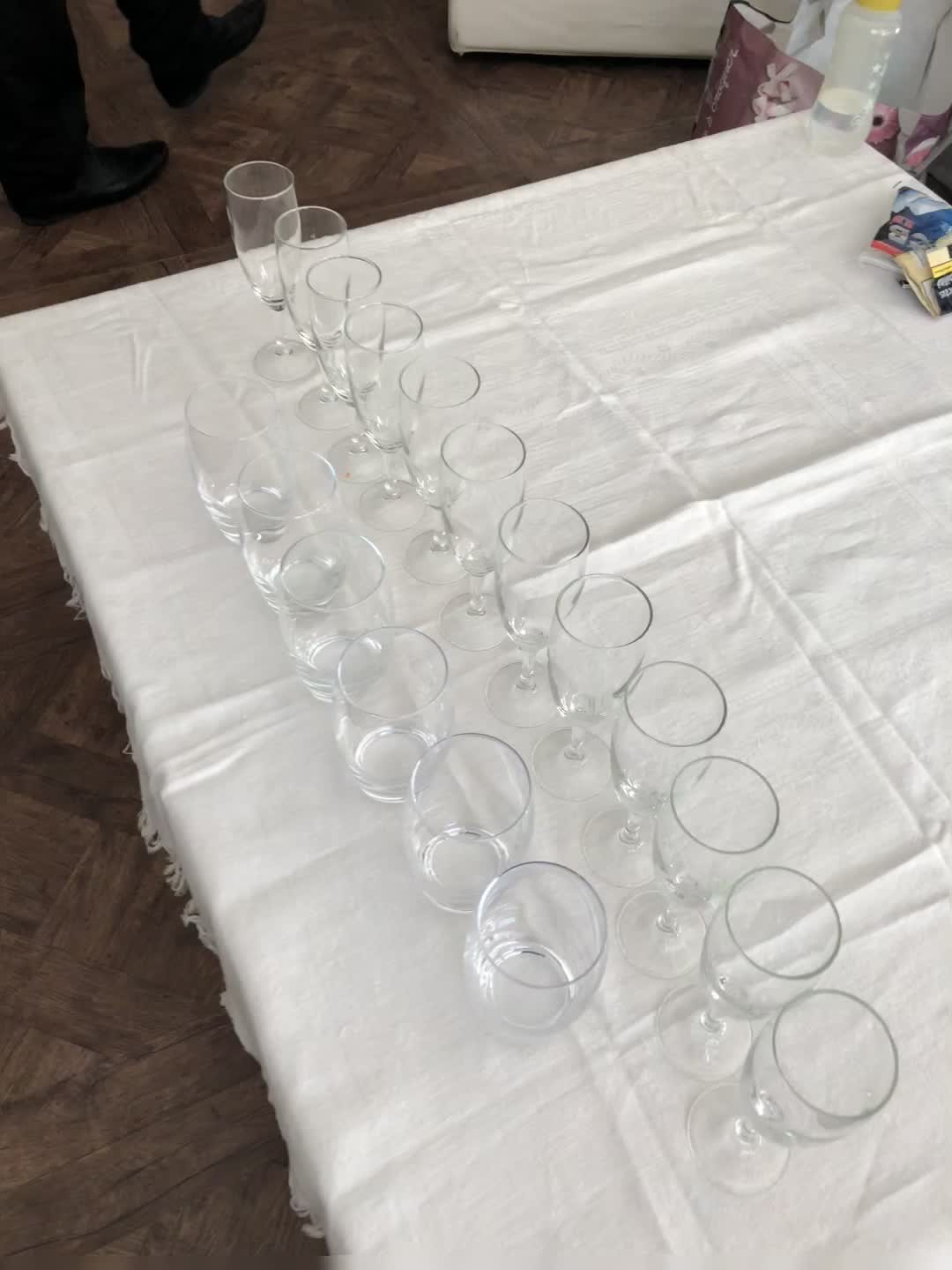This indoor digital photograph captures an overhead view of a table meticulously set for a gathering, possibly a party or a holiday like Passover. The square table, covered with a recently unfolded white tablecloth displaying noticeable creases and frills along the edges, is positioned on a floor with an intricate wood grain or mosaic pattern featuring shades of light and dark brown arranged in a zigzag pattern.

At the center of the image, approximately 16 glasses are organized for the event: 10 elegant wine goblets in the background and 6 shorter water glasses in the foreground. In the upper right corner of the table, there's a clear plastic bottle, partially filled with a clear liquid, accompanied by a couple of indistinct items in blue and yellow plastic baggies. A rose-colored bag, potentially holding a baby or juice bottle, is also partially visible nearby.

In the top left corner of the image, a person wearing black dress pants and shoes is slightly obscured, adding a subtle human element to the scene. The overall composition, combined with the detailed setting and peripheral items, suggests preparations for a warm and thoughtful gathering.